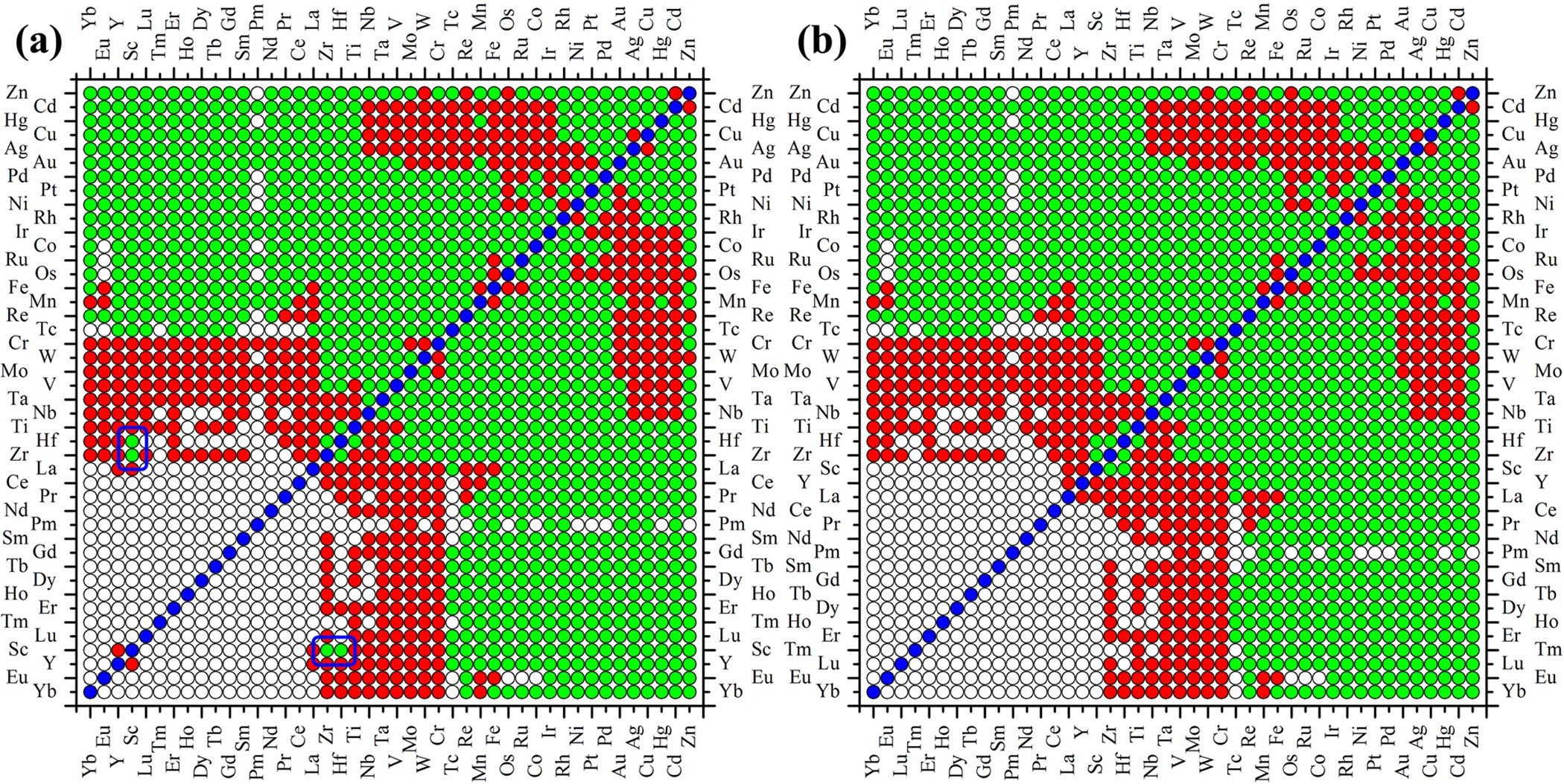The image features two side-by-side, horizontally-aligned square tables labeled A on the left and B on the right. Each table is bordered by a black outline with ruler-like markings along the top, bottom, left, and right edges, serving as the X and Y axes. Both tables are densely populated with small circles in various colors, predominantly green, which signify distinct elements or data points. Red circles are concentrated in the lower left and upper right quadrants, while a white, somewhat squarish area also appears in the lower left quadrant of each table. Blue circles form a diagonal line that extends from the bottom left corner to the top right corner in table A, and similarly from top right to bottom left in table B. The tables include chemical symbols such as Cd, Cu, Au, Pt, Rh, Co, Os, and Mn, arranged along the vertical axes. Although both tables are visually similar, subtle differences in the distribution of green and red dots suggest slight variations in the data they present.